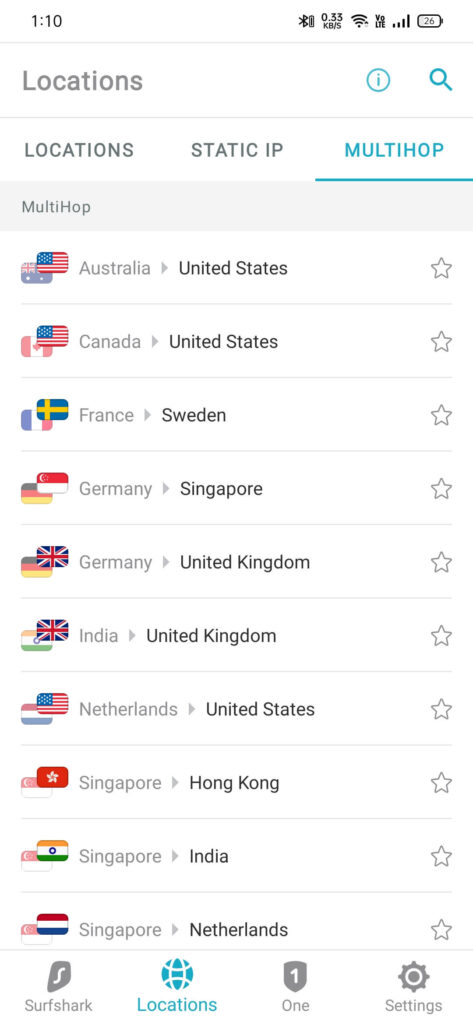The image displays a user interface with a predominantly white background. In the top right corner, there is a battery icon showing either 26% or 25% charge, alongside a Bluetooth symbol. The interface includes a prominent blue circle containing an eye and magnifying glass, suggesting a search or surveillance function. 

The screen features an underlined "Locations" header in blue, which seems to categorize various geographical options. Below this, there is an assortment of regions listed with stars next to them, including: Multi-hop, Australia, United States, Canada, France, Sweden, Germany, Singapore, United Kingdom, India, Netherlands, and Hong Kong. Each country listed has a star icon, possibly indicating a favorite or bookmarked status.

Additionally, the word "Locations" appears again at the bottom, this time placed inside a blue, globe-like oval next to a badge with the number one, which might signify a notification or an important update. The interface also has a "SurfShark" section denoted by an 'S' inside a gray oval, likely representing a VPN service. A settings icon labeled "Settings" is also present, hinting at customizable options within the interface.